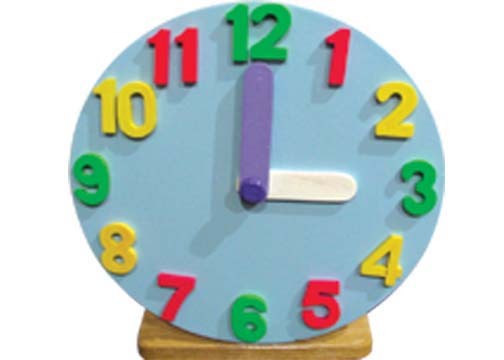This image features a children's teaching clock designed to make learning to tell time engaging and straightforward. The clock is mounted on a small, light brown, rectangular wooden base. The clock face itself is a sky-blue circle adorned with large, brightly colored numbers from 1 to 12 arranged in a clockwise sequence. The numbers are color-coded for visual appeal and easy differentiation: 1, 5, 7, and 11 are red; 2, 4, 8, and 10 are yellow; and 3, 6, 9, and 12 are green. The clock hands are distinct in color as well, with the minute hand in a vibrant purple and the hour hand in white. This setup, with its bold colors and clear design, serves as an excellent tool for teaching children how to read a clock, providing a static yet visually stimulating learning experience.